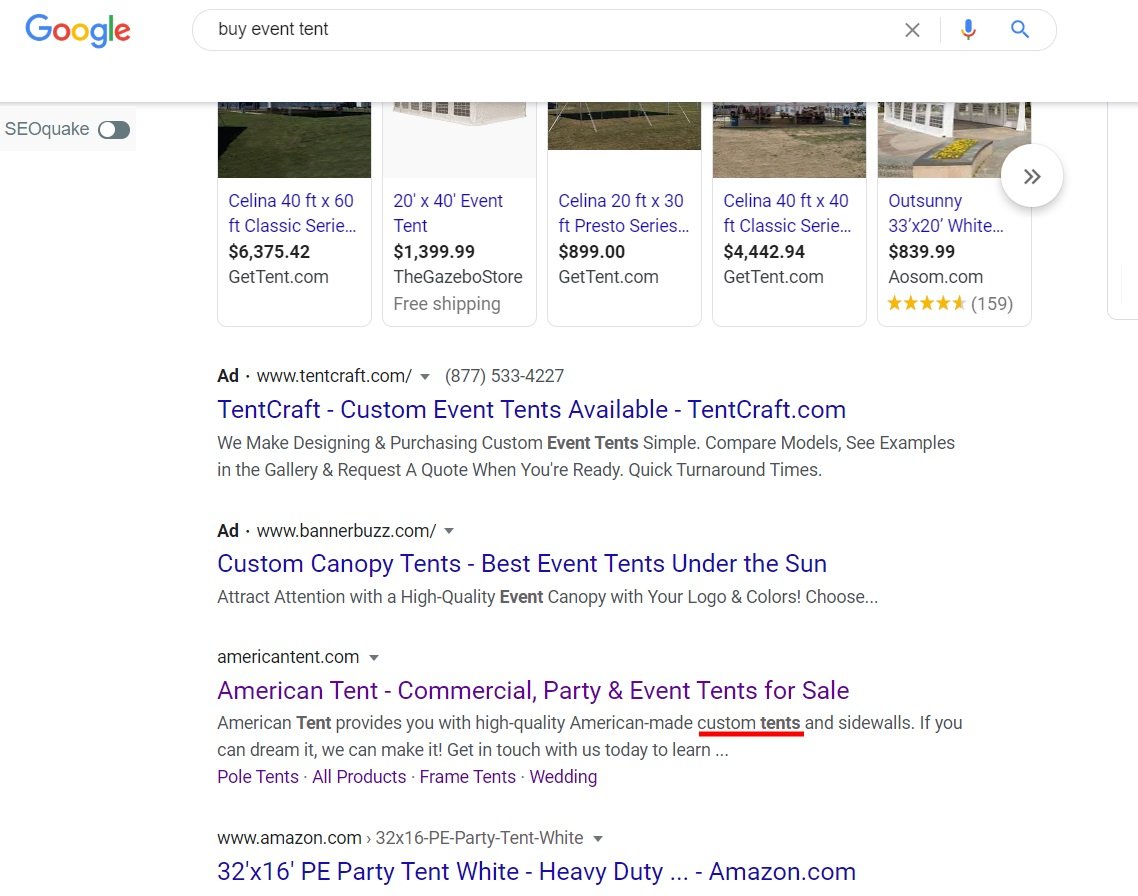The image appears to show a Google search results page for event tents. The search bar includes options like an 'X', a microphone, and a magnifying glass icon. Below the search bar, there are listings for various tents and their prices:

1. **SEL Quake Toggle Bars**: This feature is shown as turned off.
   
2. **Tents Overview**:
   - Selena 40 feet by 60 feet Classic Series: $6,375.42
   - 20-inch Reflect by 40-foot Event Tent: $1,399.99
   - Selena 20 feet by 30 feet Presto Series: $899.00
   - Selena 40 feet by 40 feet Classic Series: $4,442.94
   - Sunny 33 feet by 20 feet White: $839.99

3. **Retailer Information**:
   - Listed retailer: Awesome (aosom.com) with a rating of 4.5 stars based on 159 reviews.

4. **Suggested Websites**:
   - TentCraft (custom event tents, event tents available at tentcraft.com)
   - Custom Canopy Tents
   - Best Event Tents Under the Sun 

Each listing provides detailed measurements, series names, and pricing, offering a variety of options for event organizers looking to purchase or compare event tents. This curated search result is designed to assist in finding the most adequate tent setups for different event needs.